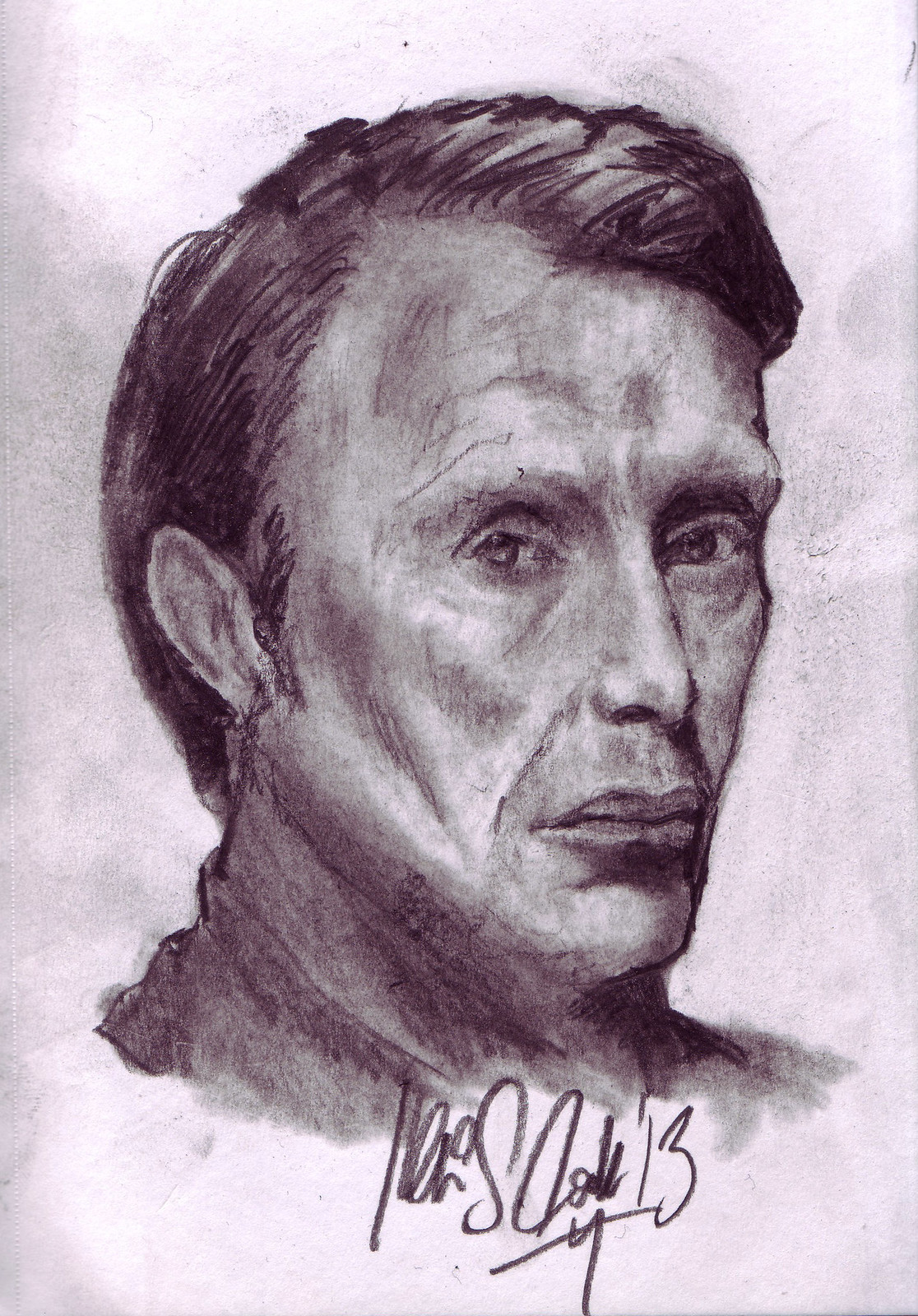This image is a detailed photograph of a pencil sketch depicting a middle-aged man, possibly aged between 45 to 55 years. The drawing is centrally focused on the man's face, with just enough of his shoulders visible before the image cuts off at the bottom. The background of the sketch consists of plain white paper, marred by some gradient gray shading and smudges, suggesting areas where the drawing might have been rubbed off.

The man, characterized by a slightly receded hairline and dark, sleek hair parted to the side, has delicate features with faint eyebrows, big eyelids, and small, deep-set eyes looking slightly off-center. His nose is small and slender, while his lips are pouty and wide, enhancing the gaunt appearance of his hollowed cheekbones and visible nasolabial folds. Dark shadows emphasize his thick neck and the area beneath his chin, adding a somber tone to his overall expression.

The artist has skillfully used different pencil strokes to create various textures and shades, especially noticeable in the detailed hair and the dark, shadowy contours around the man's face. Despite the smudges and shading in the background, the focus remains sharply on the subject’s face, highlighted by the contrast between light and dark areas.

At the bottom of the sketch, a signature in stylized cursive is visible, followed by the number '13.' However, the signature is too illegible to discern the artist's name.